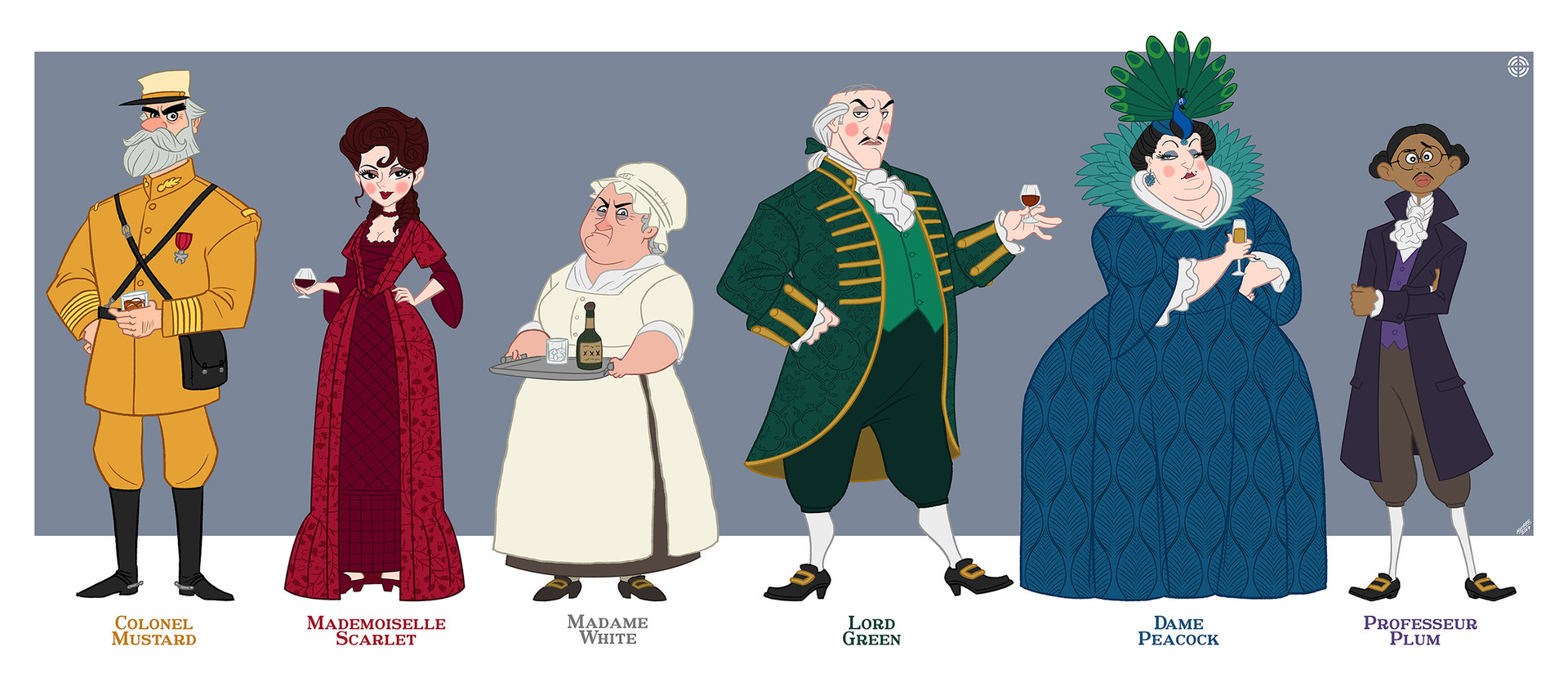A detailed illustration of six cartoon characters resembling figures from the game "Clue." From left to right, we see:

- **Colonel Mustard**: An elderly man in a light brown uniform, a light yellow hat, black boots, and a gray beard. He holds a glass in front of him. Below him, the name "Colonel Mustard" is displayed.
- **Mademoiselle Scarlet**: A woman in a long scarlet gown with dark, curled hair over her forehead. She is holding up a wine glass. The name "Mademoiselle Scarlet" is noted beneath her.
- **Madame White**: An older, stout woman dressed in a light yellow (white in some descriptions) dress and a matching hat. She holds a tray with a glass on it. Below her, it reads "Madame White."
- **Lord Green**: A bald man in a green suit with dark green, fluffy pants, and yellow detailing. He has white stockings, fancy shoes, and holds a wine glass. His name "Lord Green" is written underneath.
- **Dame Peacock**: A very large woman in a big blue dress with a ruffled collar and peacock feathers extending from her head. She holds a wine glass. Her name "Dame Peacock" is written beneath her.
- **Professor Plum**: A dark-skinned individual with black glasses, wearing a purple long coat and brown pants. Below him, it says "Professor Plum."

All characters are standing on a white surface against a light violet (or gray) background.